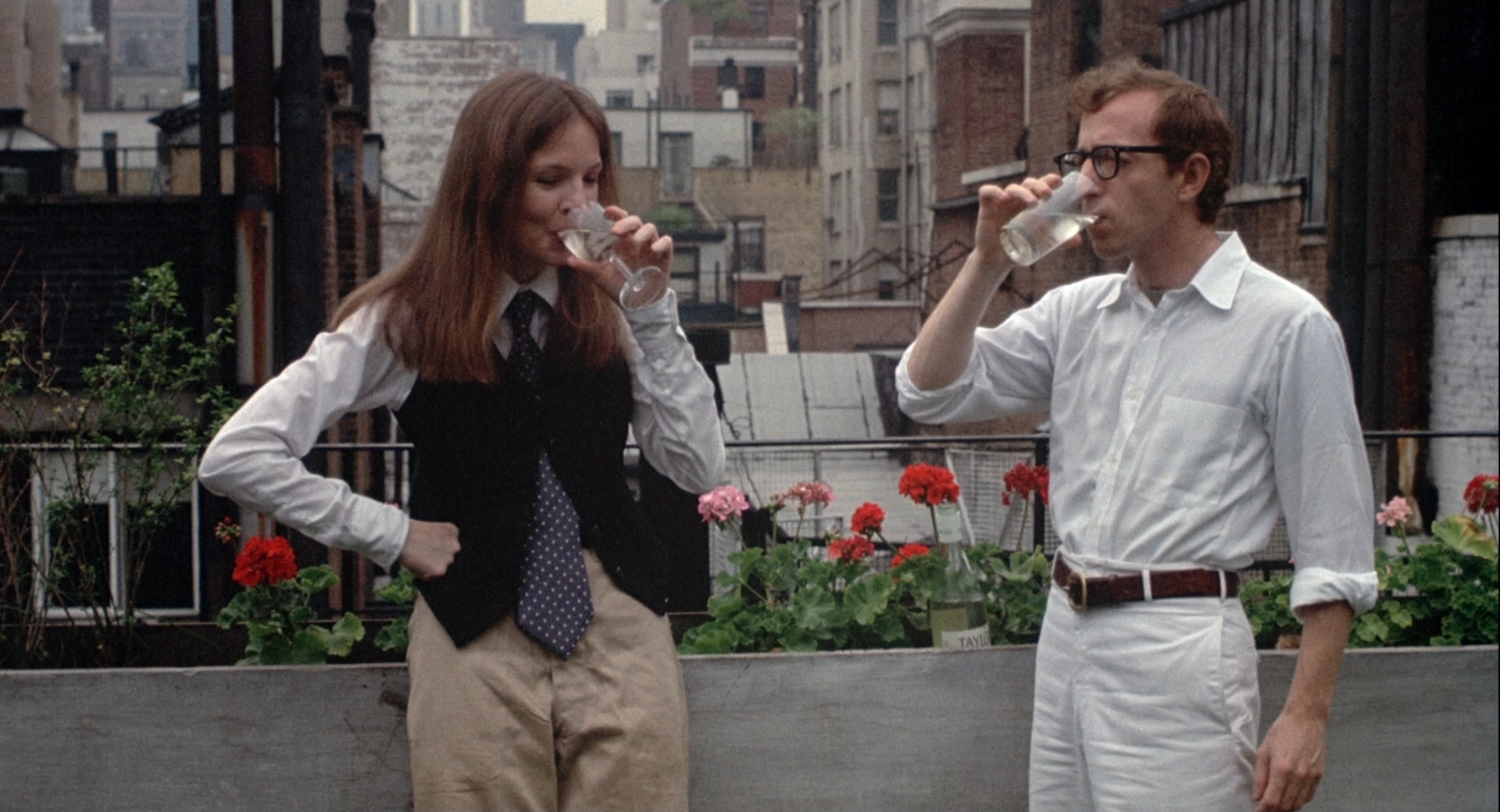In this still shot from a Woody Allen movie, both Woody Allen and Diane Keaton are standing on a rooftop in New York City. Woody Allen, characterized by his short brown hair and glasses, is on the right side of the image. He is casually dressed in a white button-up shirt with rolled-up sleeves, white bottoms, and a brown belt, and he is holding his arm up as he drinks from a glass of water. On the left, Diane Keaton is seen in her signature attire: beige slacks, a white shirt, a black vest, and a striking navy blue tie with white polka dots. She has shoulder-length brown hair and is holding a wine glass to her lips. The backdrop reveals the internal buildings of Manhattan rather than its iconic skyline. Red flowers adorn the ledge of the building, adding a touch of color to the urban setting.